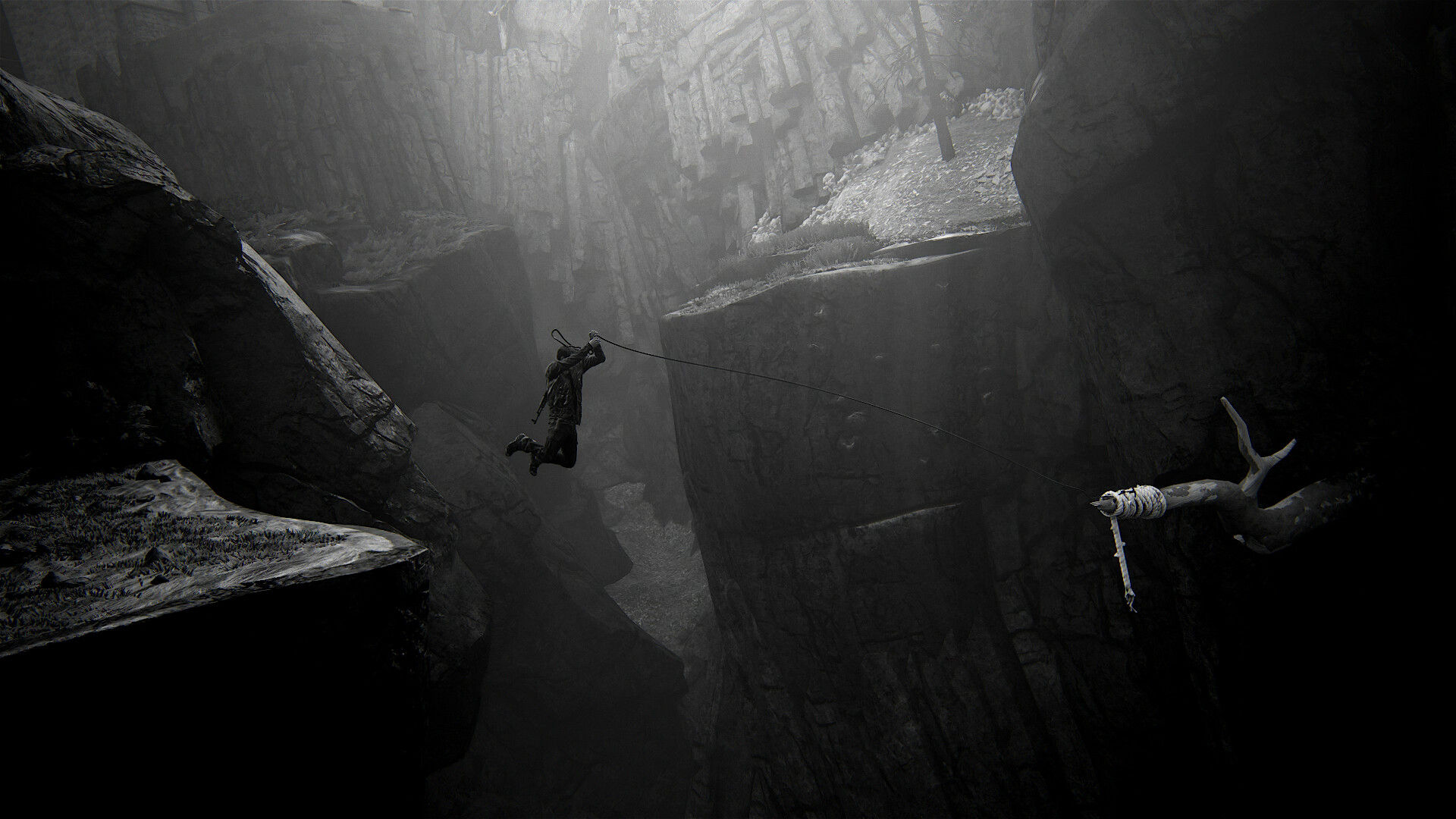In this striking black-and-white photograph, towering cliff faces loom close together, creating a sheer, precipitous drop between them. A man, seemingly suspended in midair, clings to a length of rope securely fastened to one of these rugged rock surfaces. He is attired in black pants and appears to be barefoot, wearing a long-sleeved shirt and carrying a backpack. The image captures the precarious nature of his position, emphasizing the dramatic tension of the scene. In the foreground, a flat, slippery-looking rock platform juts out, appearing muddy and dangerous, echoing the perilous drops of the surrounding cliffs. The photograph's high contrast accentuates the textures and gravity of the landscape.